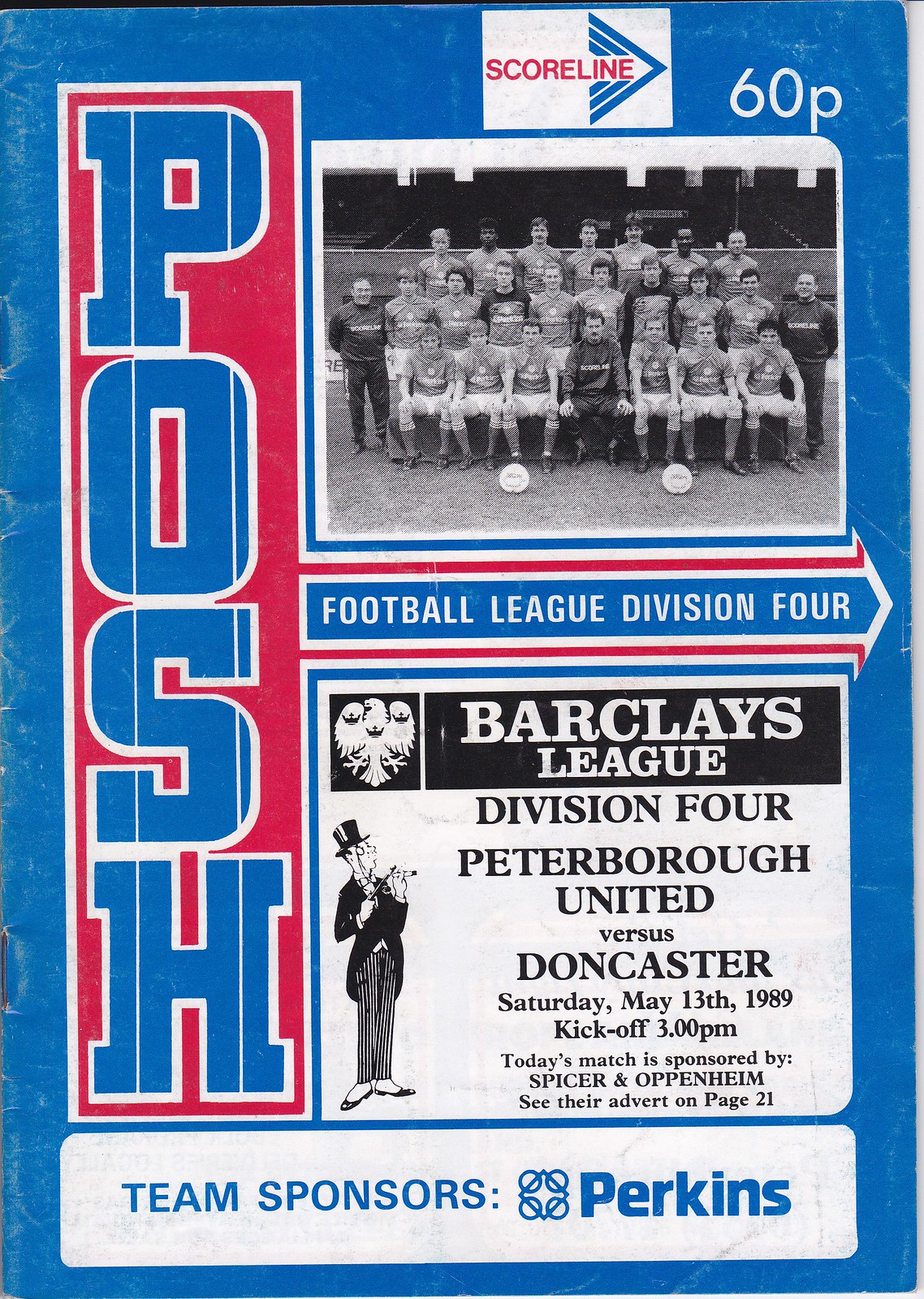This vintage program cover for an English Football League Division 4 match features a predominantly blue background with accents of red text and blocks. On the left side, the word "POSH" is prominently displayed in a vertical orientation. At the top, a logo reads "Scoreline." The centerpiece of the cover is a black-and-white photograph of approximately 22 football players positioned in three rows on a field, with two soccer balls placed in front of them. 

The program details a match between Peterborough United and Doncaster, scheduled for Saturday, May 13, 1989, with a kickoff time of 3:00 PM. Below the photograph, it reads, "Football League Division 4" and "Barclay League Division 4." Additional text notes that today's match is sponsored by Spicer and Oppenheim, with further reference to their advertisement on page 21. At the bottom of the cover, the team sponsor "Perkins" is credited. The cost of the program is listed as 60 pence, indicated by "60P" in the top right corner.